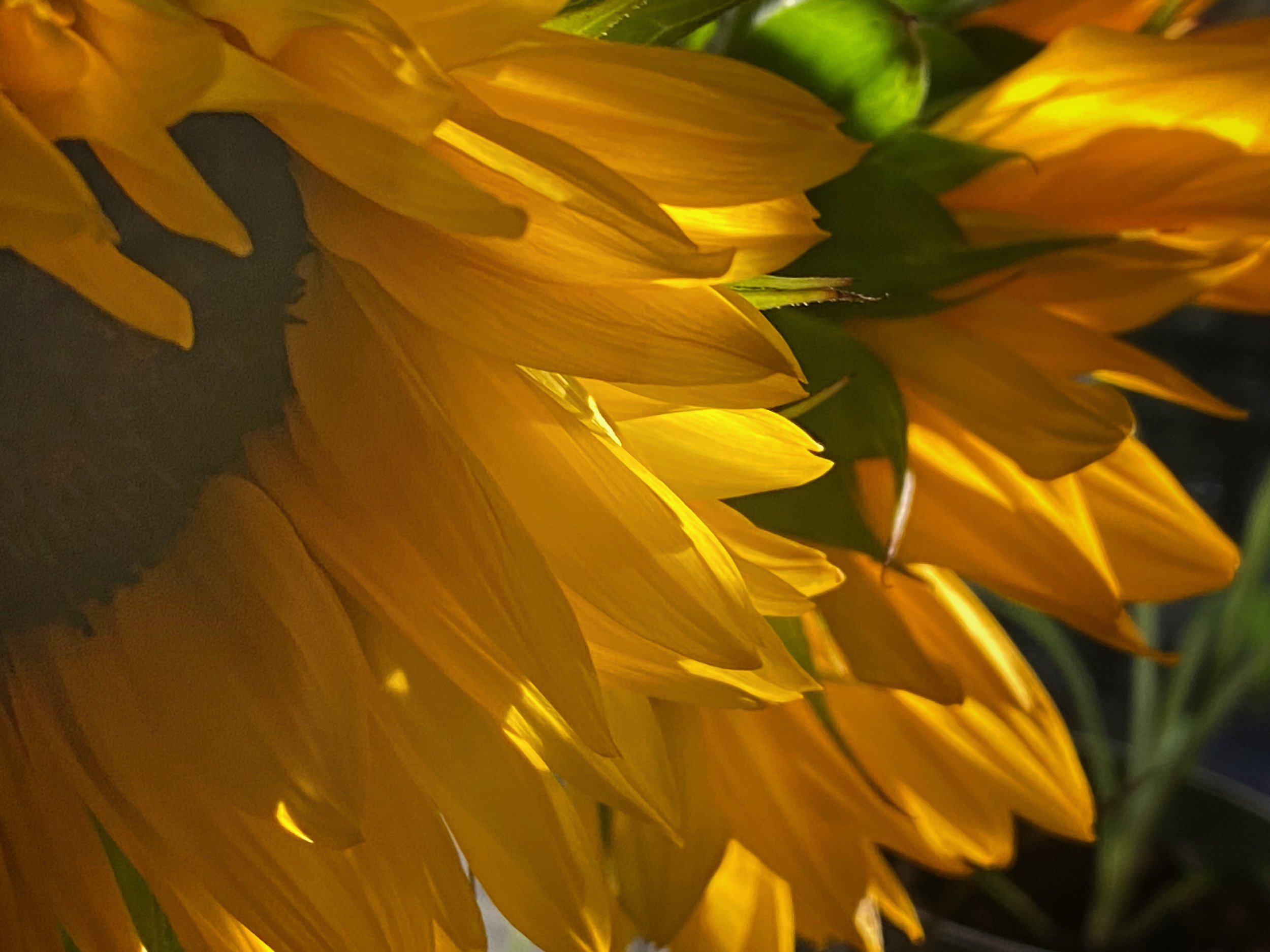This photograph is a vibrant and detailed close-up of several large sunflowers, primarily focusing on one striking sunflower located in the upper left-hand corner. The intricate details of the sunflower are beautifully captured, with the deep, dark brownish-orange center dominating the left side of the image. Surrounding this center are an estimated 30 to 40 densely-packed yellow petals, their rich and varied shades illuminated by the soft sunlight, which appears to evoke an afternoon or dusk setting. Behind the primary sunflower, the composition reveals green leaves and additional yellow petals, indicative of more sunflowers, though their centers remain out of view. The light piercing through the petals and reflecting on the stems enhances the vivid, crisp textures, creating a scene that feels almost tangible. The sunflowers seem to bend slightly, as if swayed by a gentle breeze, adding a dynamic feel to this sunlit field.